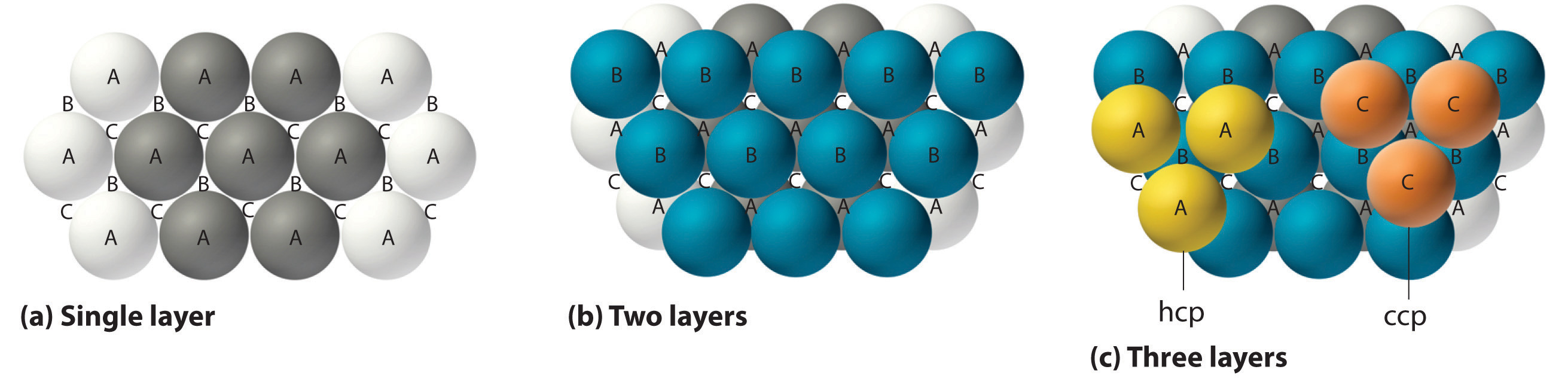The image is a detailed chemistry illustration divided into three parts, each demonstrating a different layered structure of spheres. The first part, labeled "A - single layer," consists of white and gray spheres, all marked with the letter "A." The second part, "B - two layers," adds a second layer of blue spheres labeled "B" on top of the white and gray spheres. The third part, "C - three layers," includes a third layer composed of three yellow spheres labeled "A" and three orange spheres labeled "C," in addition to the previous white, gray, and blue spheres. The labels HCP and CCP are used to describe certain groups of spheres, with HCP associated with three yellow spheres labeled "A" and CCP related to three orange spheres labeled "C." This appears to be a detailed visual explanation of a fundamental chemistry concept, potentially illustrating different atomic or molecular structures across the layers.